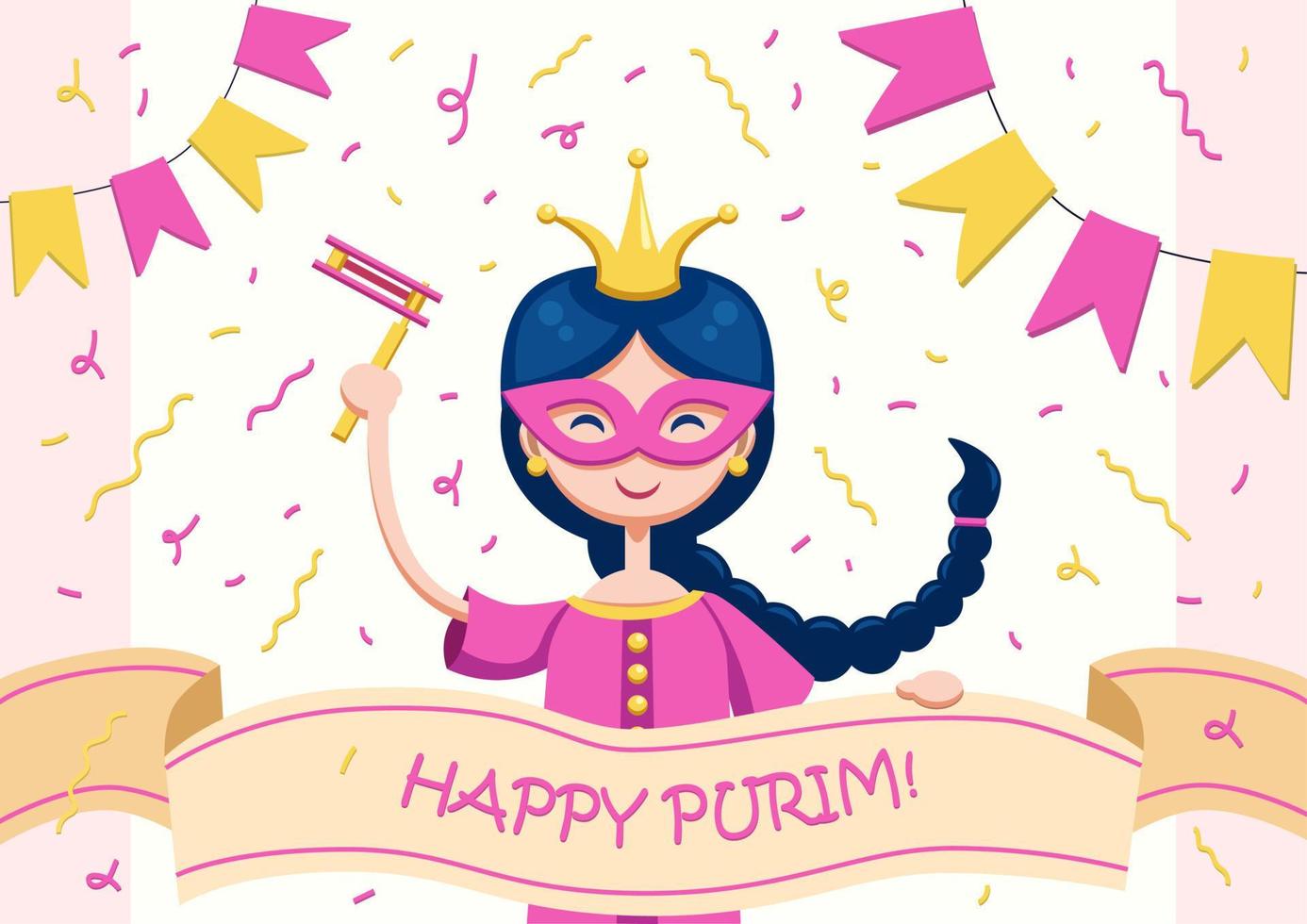This lively and detailed illustration captures a festive Purim celebration. At the center is a cheerful girl wearing a pink masquerade-style mask and a golden jester cap with three spikes, each topped with a small ball. Her dark bluish hair is intricately braided, curving behind her and up towards the sky. She is clad in a pink shirt adorned with golden buttons and matching gold earrings. In her right hand, she swings a wooden party favor that makes a ratcheting noise.

The girl holds up a tan banner across the bottom of the image that reads "Happy Purim" in purple letters. The overall scene is enriched with pink and yellow confetti showering down, enhancing the festive vibe. The background is predominantly white, framed on the sides with pink borders. Additionally, there are flag banners featuring alternating pink and yellow flags hanging in both upper corners, adding to the celebratory atmosphere.